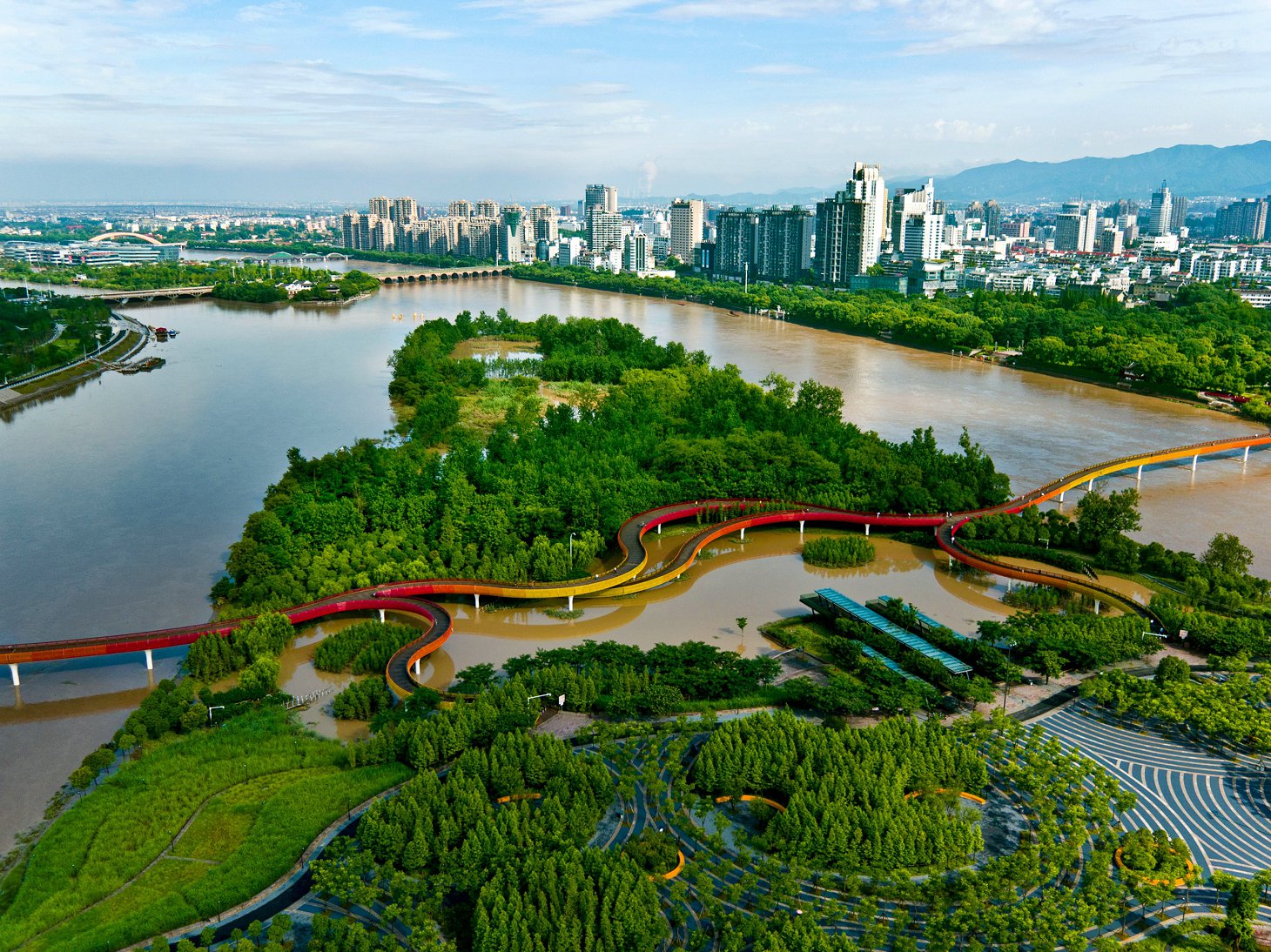This aerial, wide-angle image captures a vibrant cityscape in the background, characterized by tall, white buildings lining the skyline. In the foreground, a lush, green island bisects a large river that forks into two paths. The island features a finely trimmed, manicured garden area in the bottom left corner, giving it the appearance of a city park. A distinctive red and yellow winding walking bridge spans the river, crossing the island and reconnecting both sides of the waterway. The bridge has multiple exits leading onto the island, which also houses a brown pond and several long blue buildings. Towards the far distance in the upper right corner, a mountain range lines the horizon, adding to the scenic backdrop. Additionally, there is a car bridge over the water and potentially a small dam discernible at the head of the river. The image is highly detailed, capturing the bustling energy and complex layout of the urban setting from a bird's eye view.